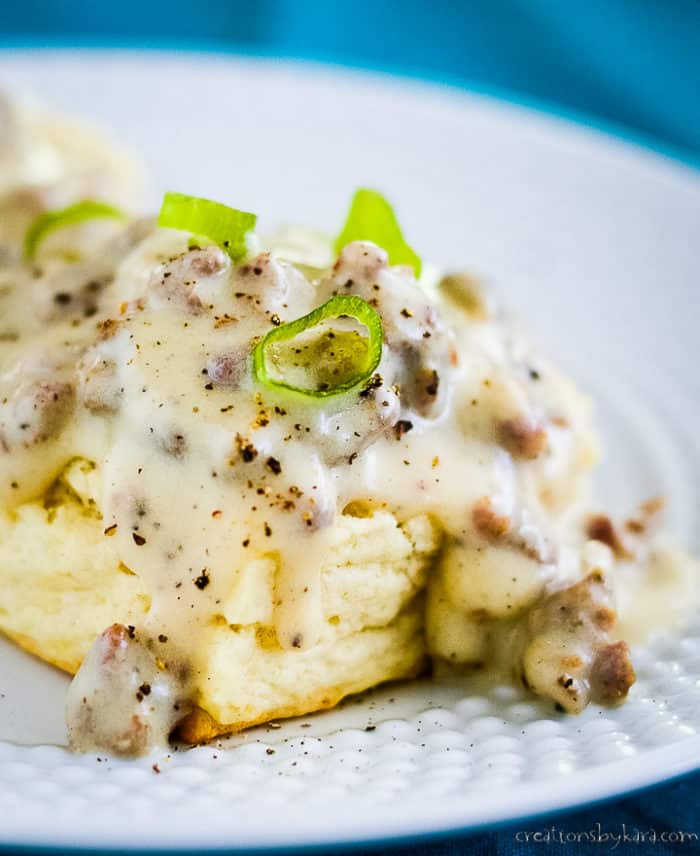The image shows a close-up photograph of a dish that appears to be biscuits and gravy, a classic American breakfast. The food is served on a white plate with a textured, hobnail design around the rim and a subtle blue rim at the very edge. The plate sits on a blue background, likely a blue tablecloth. In the center of the plate is a large, square biscuit that is crusty and brown on the outside, indicating it has been well-baked. The biscuit is split open, revealing a flaky and rich white interior. The biscuit is topped with a thick, creamy white gravy that contains visible chunks of browned sausage. Garnishing the dish are chopped green onions, adding a fresh splash of color, and a sprinkling of coarse ground black pepper. Text on the bottom of the image reads "creationsbycara.com," likely crediting the creator or photographer of this appetizing dish.